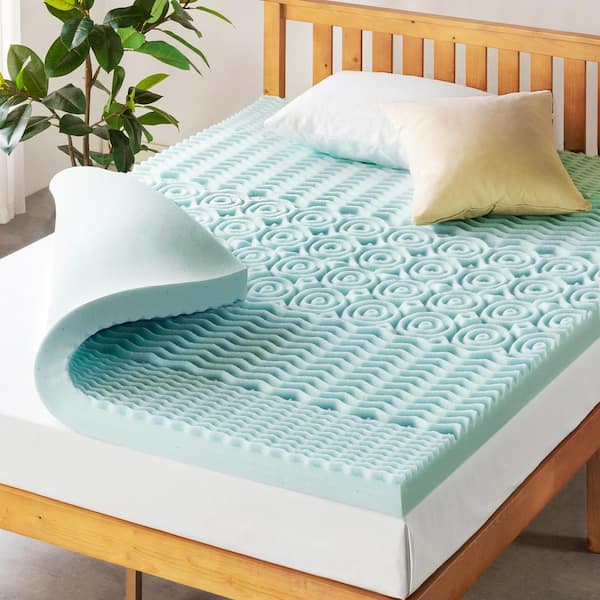This is a detailed color photograph, likely intended for marketing a mattress or mattress topper, featuring a wooden bed frame topped by two distinct layers. The upper layer is a blue latex or foam mattress topper, about six inches thick, adorned with wave patterns and circular designs, indicating its density and flexibility. One corner of this topper is deliberately folded up, demonstrating its pliability. Beneath it lies a thicker, white mattress or box spring. Two pillows without covers rest at the head of the bed, which is diagonally positioned as the main focus of the image. A tall, green plant in a planter adds a touch of nature to the scene, complementing the partial view of a curtain. The overall aesthetic and composition resemble a standard product photo, similar to those found on Amazon.